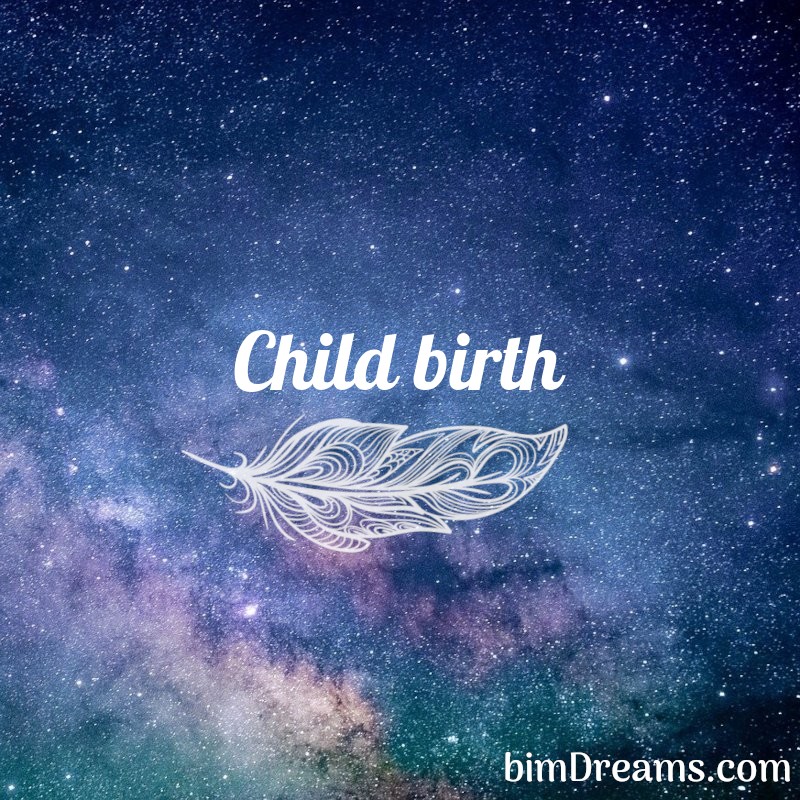The image showcases a captivating night sky with a dark blue backdrop filled with an array of white speckled stars, creating an awe-inspiring celestial scene. The upper part of the image is predominantly dark blue, speckled with various sizes of white dots depicting stars and larger star formations. In the lower portion, the sky transitions into a mesmerizing blend of purplish-pink hues, resembling ethereal clouds interwoven with the starry expanse.

At the center of the image, the word "childbirth" is prominently displayed in bold, white, cursive text. Positioned directly beneath this word is a delicate, white feather. The feather is detailed, with its stem on the left, gracefully extending to the right, featuring an intricate swirled pattern on its surface.

In the bottom right corner of the image, the website "BIMdreams.com" is inscribed in crisp white letters, providing a subtle yet clear branding element. The image as a whole harmonizes the celestial beauty of a starry night with the gentle symbolism of childbirth, elegantly conveyed through the feather and artistic cloud-like formations.